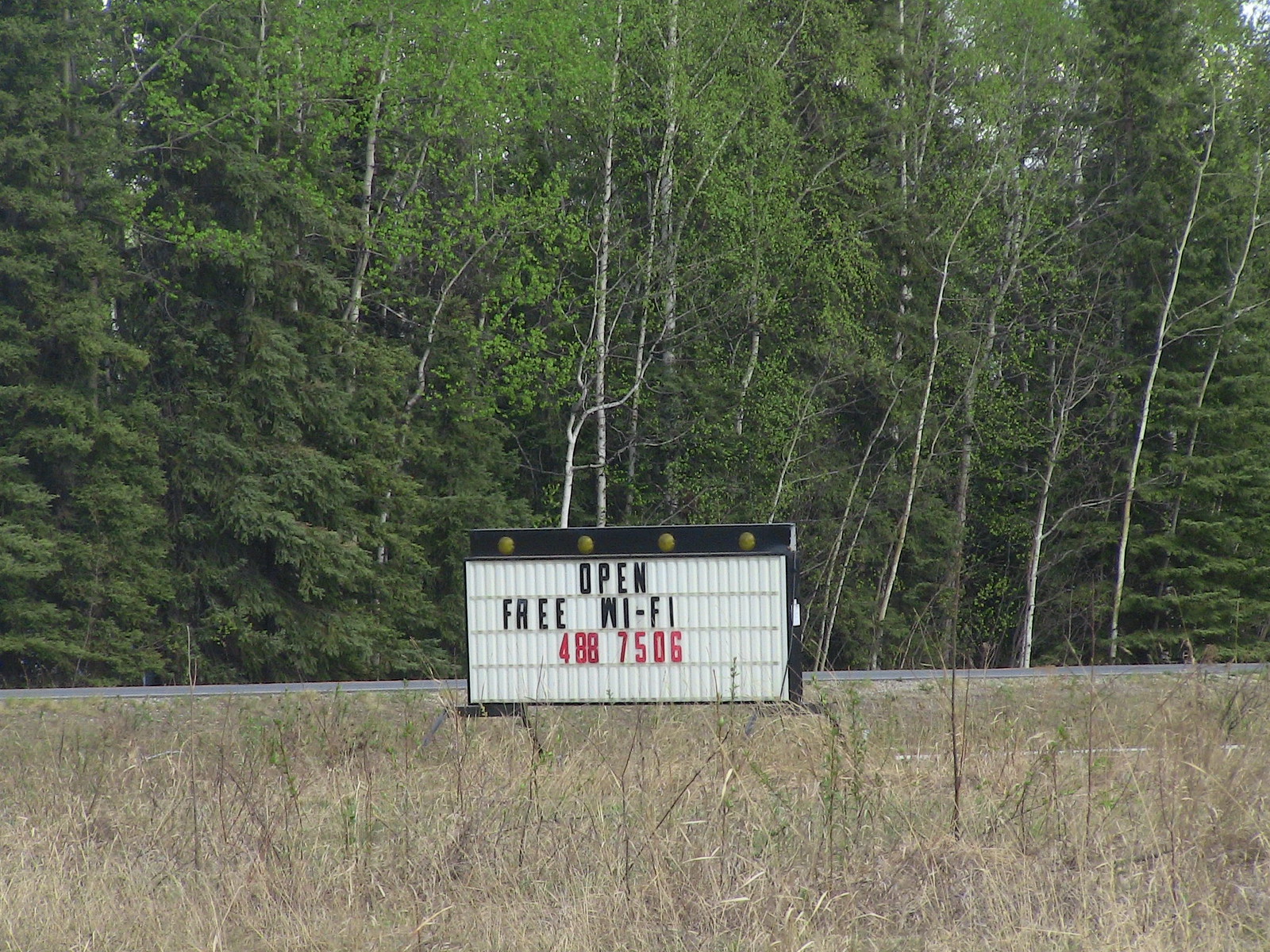The photograph captures an outdoor scene dominated by nature and a solitary roadside sign. The upper two-thirds of the image are filled with a vast expanse of tall, diverse trees reaching towards the sky. Below this dense canopy lies a quiet road, marked by a white line along its shoulder, creating a clear division between the asphalt and the wild growth beside it. Prominently positioned near the road’s edge stands a rectangular advertising sign. This sign, in a field of dried weeds, features a white background with a black border at the top, adorned by four greenish lights. The main body of the sign displays the text "Open 3Y-F5-488-7506," providing a stark, utilitarian message amidst the natural, untamed surroundings.